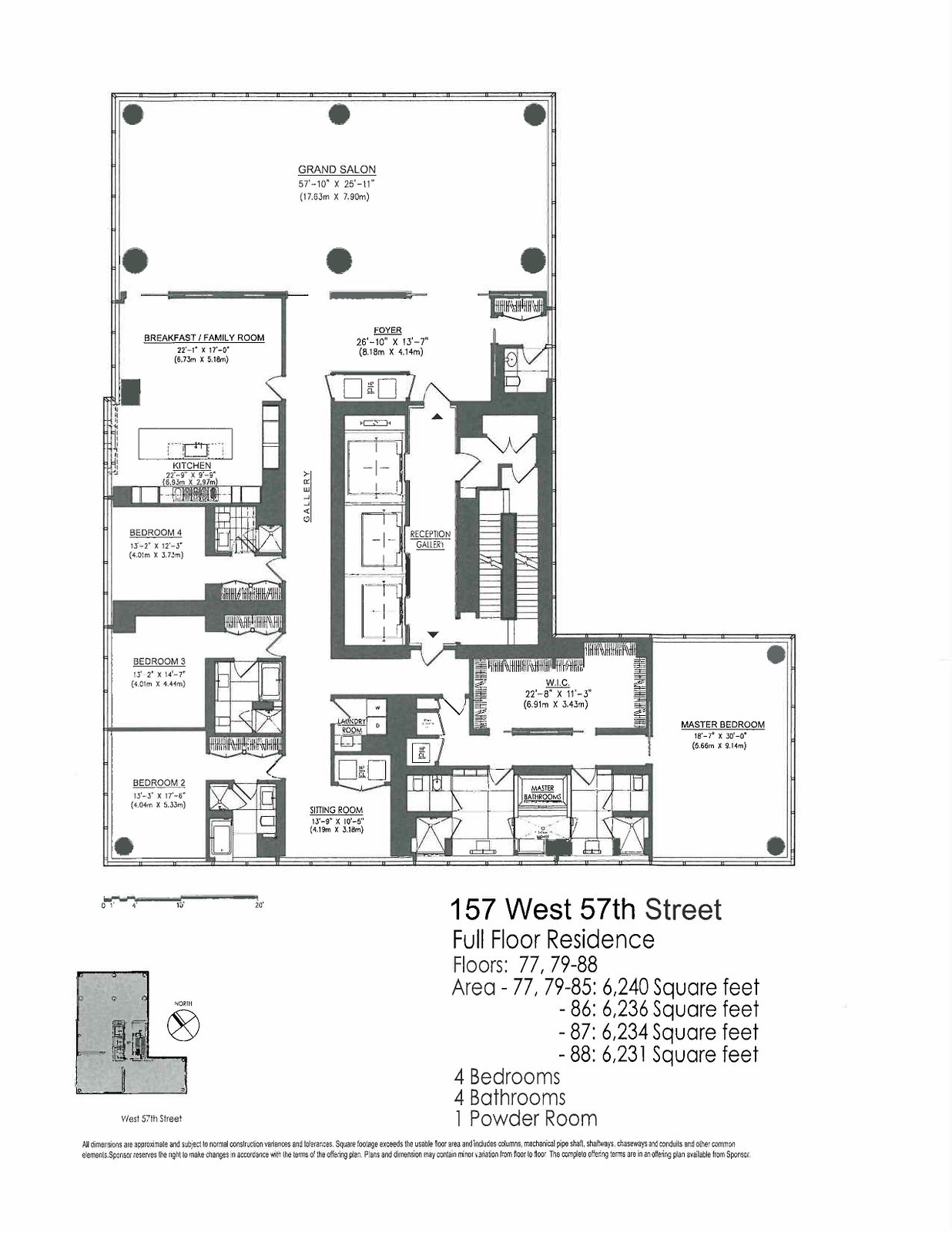This detailed floor plan of a full floor residence at 157 West 57th Street spans the 77th, 79th-88th floors, with varying square footage: Floor areas from 77, 79-85 cover 6,240 square feet, floor area 86 is 6,236 square feet, floor area 87 is 6,234 square feet, and floor area 88 is 6,231 square feet. The residence features four spacious bedrooms, four full bathrooms, and one powder room.

An overhead scale, whose exact measurements are not clearly readable, measures roughly one inch to ten feet. At the upper section of the schematic, there is a grand salon, complete with specific measurements. Adjacent is a combined breakfast and family room with an adjoining kitchen. Near the kitchen area, you'll find the foyer which houses a closet and a restroom.

Central to the layout is a gallery, branching off to bedroom four, furnished with its own full bathroom and closets. Progressing downward to the middle of the residence is bedroom three, also accompanied by a private bathroom and closets. Towards the lower end of the schematic, bedroom two mirrors this setup with an en-suite bathroom and closets. 

Continuing straight through the gallery, you encounter a sitting room and additional closet space. Nearby is the laundry room, conveniently located towards the center. The reception gallery, marked centrally in the floor plan, highlights three doorways leading to unspecified spaces. To the right, a set of stairs is indicated.

Finally, at the schematic's tail end, a doorway ushers you to the master suite. This section includes the master bedroom, a spacious walk-in closet, and a luxurious master bathroom, completing the elegant and meticulously detailed floor plan of this high-floor residence.